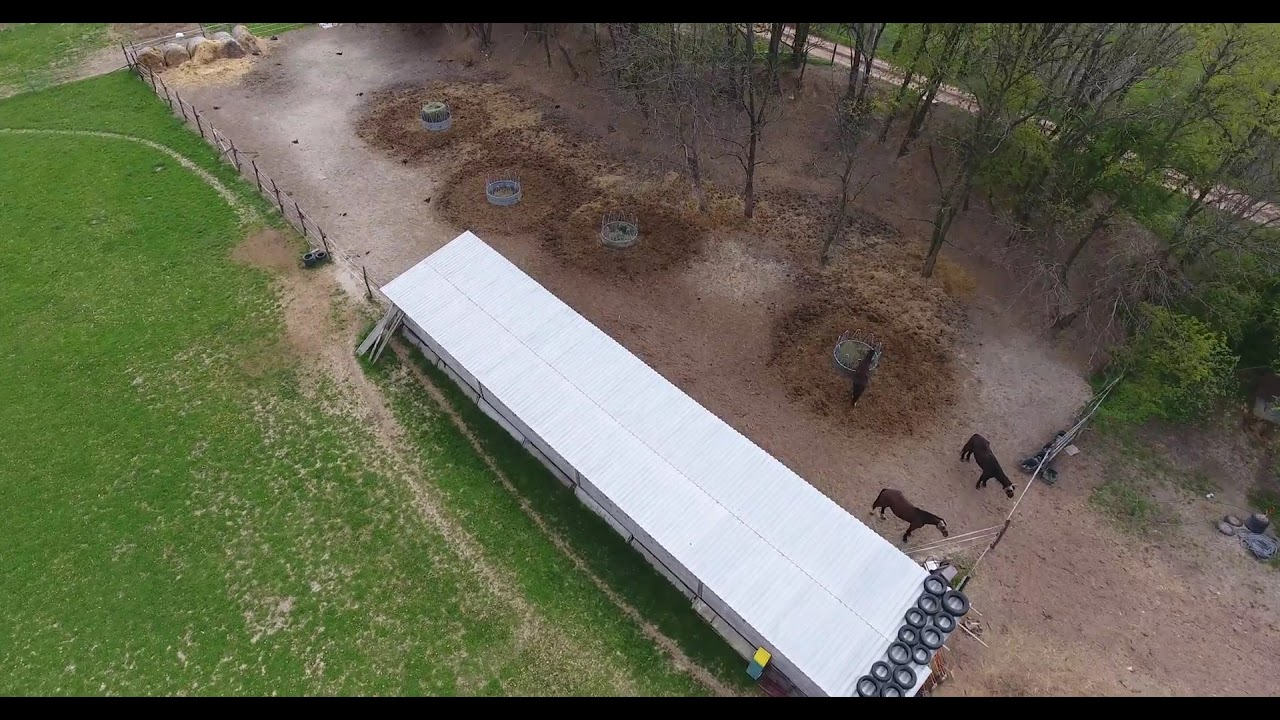This is an overhead shot of a horse farm, featuring a rectangular enclosure divided into separate areas of grass and dirt. The left side of the enclosure has patches of green grass, while the right side is primarily dirt, with some areas where the soil appears to have been disturbed, possibly for feeding or watering placements. Inside the fence, there are three brown horses standing near the right-hand side, by a large white structure that looks temporary, perhaps a horse shelter for weather protection. Behind the horses, there's a person too distant to clearly identify. Surrounding the enclosure are a few leafless and green trees, with a road visible beyond them. The overall atmosphere of the scene is gray and overcast, with no visible shadows, suggesting an overcast day.